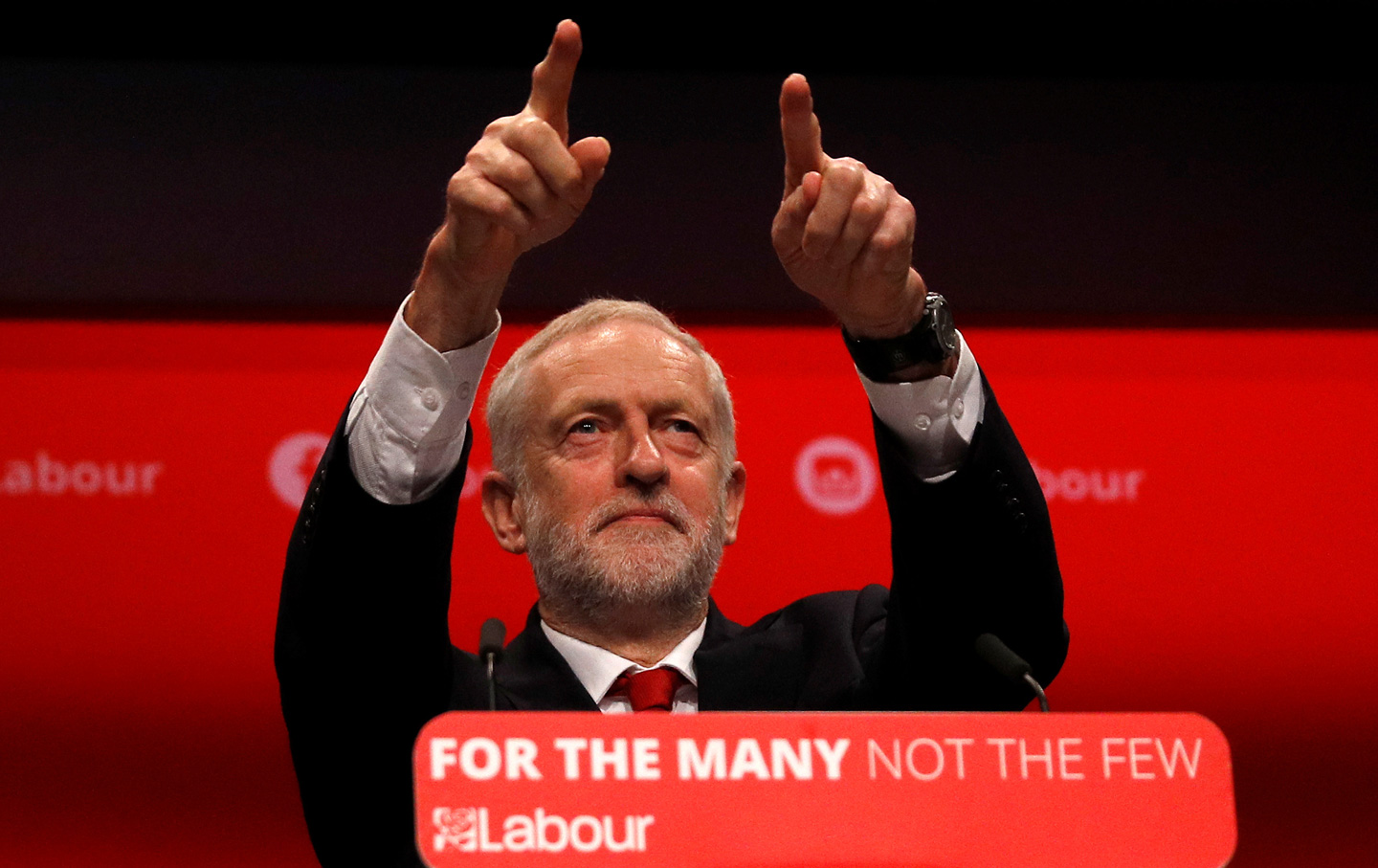The image depicts a bearded politician, possibly in his 60s or 70s, standing at a podium adorned with a prominent red sign that reads "For the many, not the few, Labour." He is dressed in a black suit, white button-down shirt, and a red tie, complemented by a wristwatch on his left hand. The man is engaged in an animated gesture, pointing upwards and outwards with his left hand. The background features a large red banner with the word "Labour" in bold white letters, and a black strap covers about a third of the upper part of the image. The setting strongly suggests that he is at a Labour Party event, likely within the UK, given the spelling of "Labour" and the party's logo. The background's vivid red color has an intense, almost rally-like ambiance. Small microphones are positioned on either side of the lectern, indicating a well-prepared speech in progress.